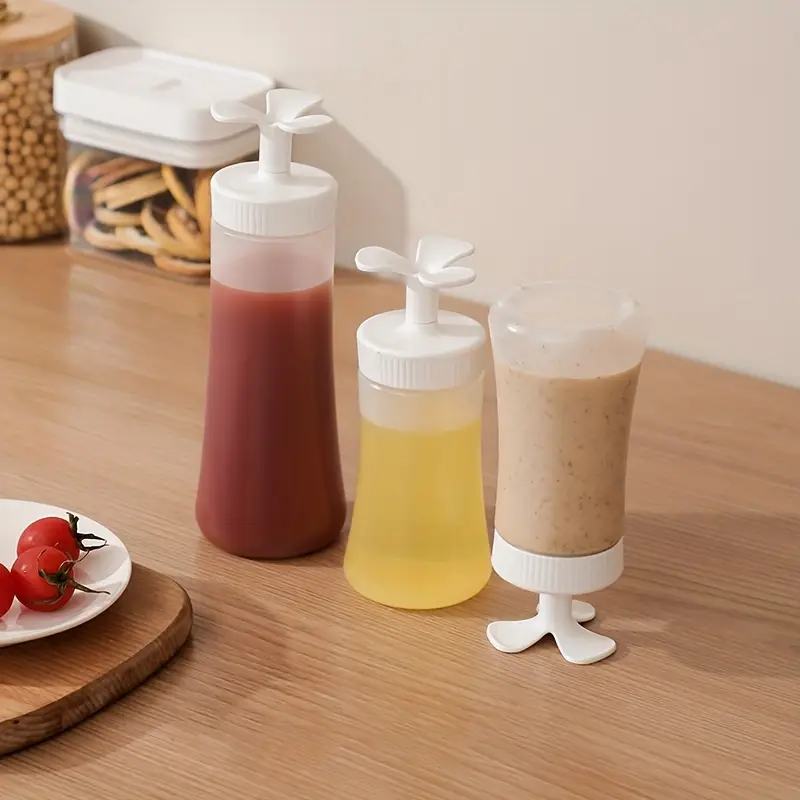This detailed close-up photograph showcases three uniquely designed condiment bottles arranged on a light-colored wooden table. Each bottle features a cylindrical shape that tapers towards the bottom, topped with a white, flower-like dispenser cap. The three petals of these dispensers are connected by a cylindrical spout. The largest bottle, positioned on the left, contains a red substance likely to be ketchup. The middle bottle, which is of medium size, is filled with a yellow liquid, possibly oil. The smallest bottle on the right is upside down, resting on its flower petal spout, and filled with a light brown substance speckled with black, suggesting it might be a type of salad dressing.

To the left of these condiment bottles, a wooden cutting board or serving tray holds a ceramic plate topped with three deep red cherry tomatoes, some of which have wilted green leaves. In the background, slightly blurred, there's a cookie jar with a white lid, which contains thin, light brown cookies. Beside this, another glass container with a wooden lid holds numerous small, pea-like, light brown objects.

All of these items are set against a plain white backdrop, providing a clean and focused aesthetic to the image.